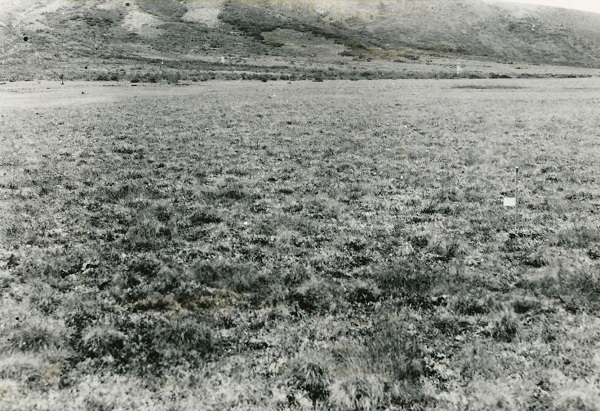The black and white photograph depicts a desolate and barren landscape, reminiscent of a scene from a long time ago. The bottom three-quarters of the image features a vast, flat field sparsely covered with grass and low-growing foliage. On the right-hand side of this flat expanse, a small pole with a tiny white flag stands out as one of the few man-made items in the scene. In the background, a row of low-growing trees or scrub brushes indicates the start of an elevation. The upper quarter of the image shows a hillside or mountain with blotches of foliage, including either very low trees or grass, interspersed with large barren areas. The hillside slopes downward on the right side, blending into a sky that introduces patches of white into the otherwise grayscale composition. No people or buildings are visible, reinforcing the impression of a barren, somewhat wasteland-like setting. The central part of the picture stands out with a denser concentration of black, while the rest of the scene features varying shades of white and gray.